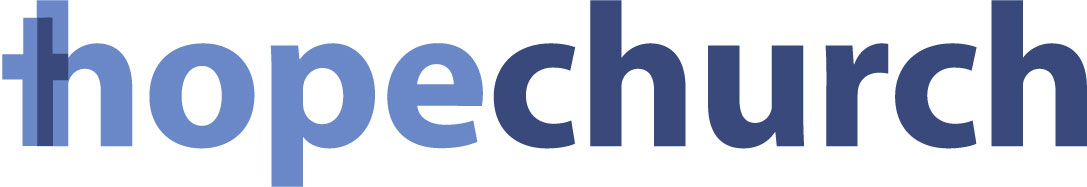The image features a minimalist logo for Hope Church, set against a pristine white background. The logo consists of large, bold text that effectively captures attention. "Hope" is rendered in light blue, while "Church" is in a darker blue. Notably, the letter "H" in "Hope" incorporates a cross halfway between the bar of the H and extending outwards, creating a unique merging of the cross and the letter's design. Additionally, the T and H are overlapping each other, blending parts of each into a darker shade at their intersection. The font used is friendly and lacks capitalization, adding to the approachable feel of the logo. Overall, this clean and simple design emphasizes the name "Hope Church," with its creative use of a cross integrated into the lettering.